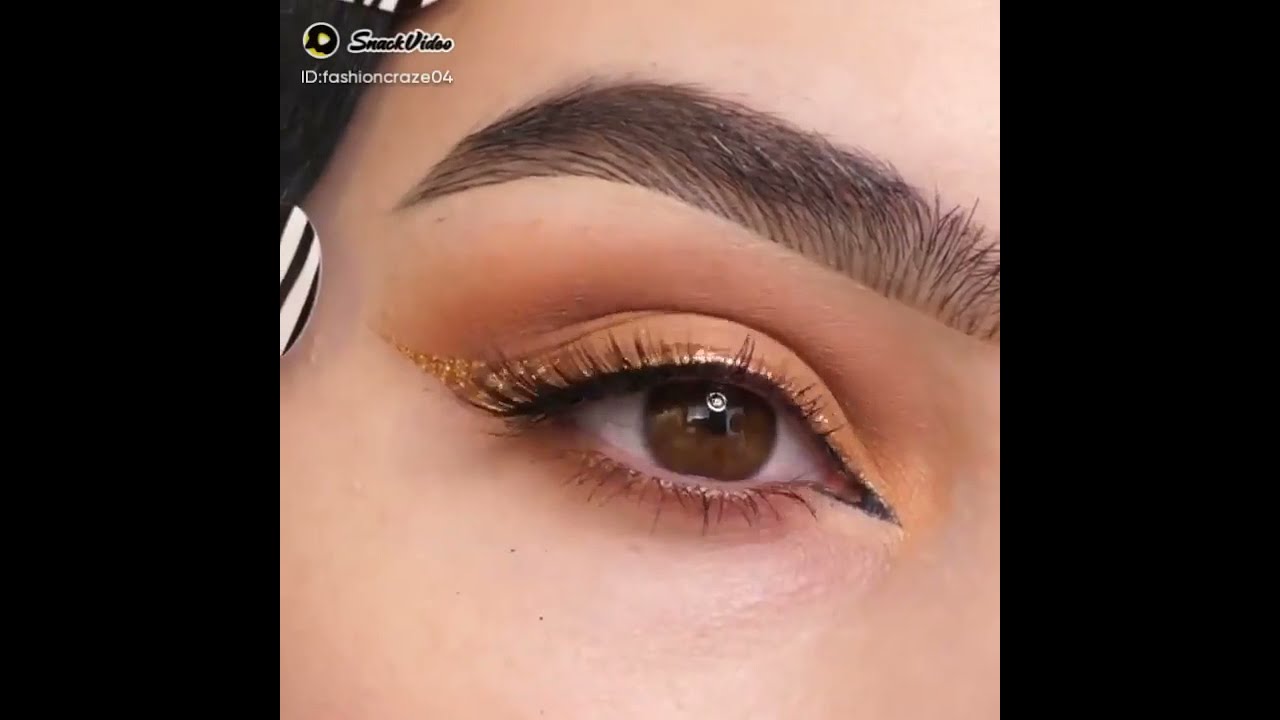This is a detailed close-up image of a woman's right eye, showcasing her beautifully done eye makeup. Her eye is a rich brown color, surrounded by brown eyelashes and dark, well-groomed eyebrows that appear strikingly styled. Her eyelids are adorned with a rich coffee-colored eyeshadow and hints of gold shimmer at the corners, topped with a glittery finish, adding to the eye's overall shine, which reflects a bright light source. Positioned in the top left corner of the image is a watermark in black text with a white outline that says "Snack Video," accompanied by an ID handle in white text that reads "FashionCraze04." To the left of the watermark, there's a logo resembling a penguin with a large nose on a yellow background within a black and white striped frame. The overall composition emphasizes the elegance of the eye makeup and the stylish presentation of the eye itself.